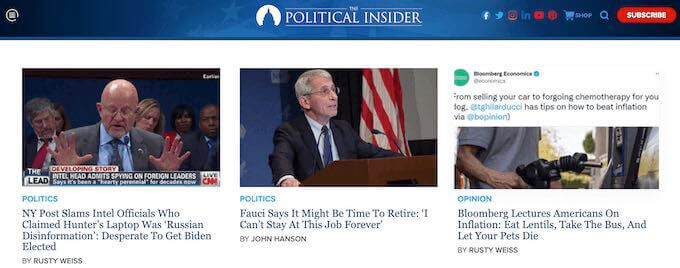This is a detailed screenshot of a website called "The Political Insider". At the top of the screen, a blue banner spans across, featuring a faint graphic of an American flag entirely in blue. The website's name, "The Political Insider," is prominently displayed in white text alongside a white circle containing the silhouette of what appears to be the Capitol building.

In the top right corner of the blue banner, there are icons for social media platforms including Facebook, Twitter, Instagram, LinkedIn, and YouTube, as well as a red circular button whose function is unclear. Next to these icons, there is a shopping cart labelled "Shop," a blue magnifying glass for searching, and a red "Subscribe" button.

Three news articles are prominently displayed on the page. The first article features an image of a man, presumably a high-ranking Intel official, speaking into a microphone while raising his hands. The headline reads, "NY Post slams Intel officials who claimed Hunter's laptop was Russian disinformation, desperate to get Biden elected," authored by Rusty Weiss, and it is filed under Politics.

The second article shows Dr. Anthony Fauci standing at a podium with an American flag in the background. The headline states, "Fauci says it might be time to retire, I can't stay at this job forever," written by John Hansen, and it is also filed under Politics.

The third article is an opinion piece originating from Bloomberg Economics on Twitter. The article discusses the impact of inflation and offers controversial advice, such as "selling your car" and "foregoing chemotherapy for your dog." The headline reads, "Bloomberg lectures Americans on inflation, eat lentils, take the bus, and let your pets die," authored by Rusty Weiss.

The background of the page is predominantly white, providing a stark contrast to the blue banner. In the upper left corner of the screen, there is a square icon circumscribed within a circle.